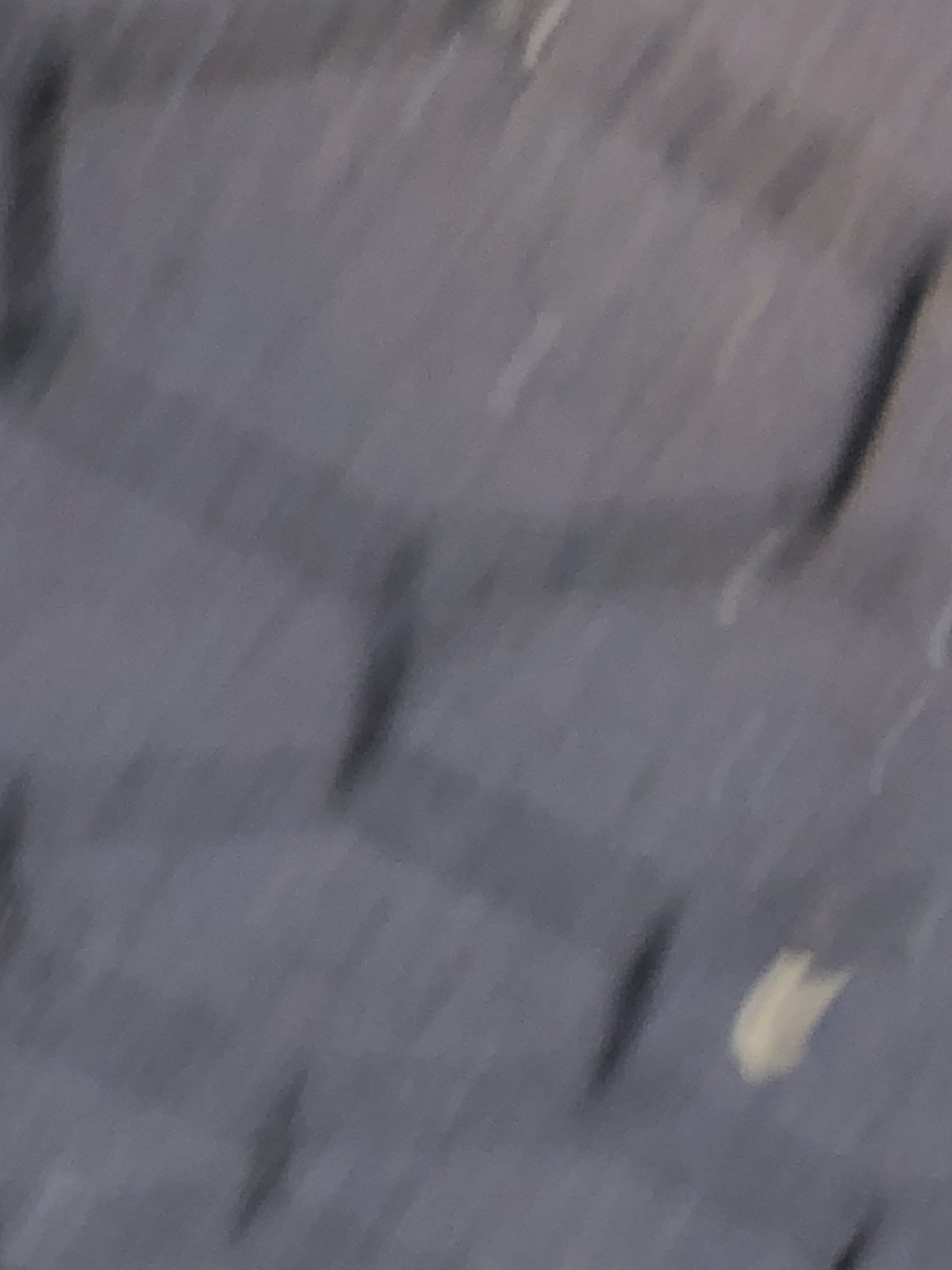This image features an extremely close-up, zoomed-in perspective of octagonal stone tiles, though the focus is notably blurred. At the center of the photograph, the thick, gray concrete tiles can be identified despite the distortion. The white mark resembling a paint stroke, situated at the bottom right corner, suggests either a stain or a scratch on the image itself. The tiles exhibit considerable unevenness, with some set considerably higher or lower than their neighboring tiles, creating a potentially hazardous surface for walking.